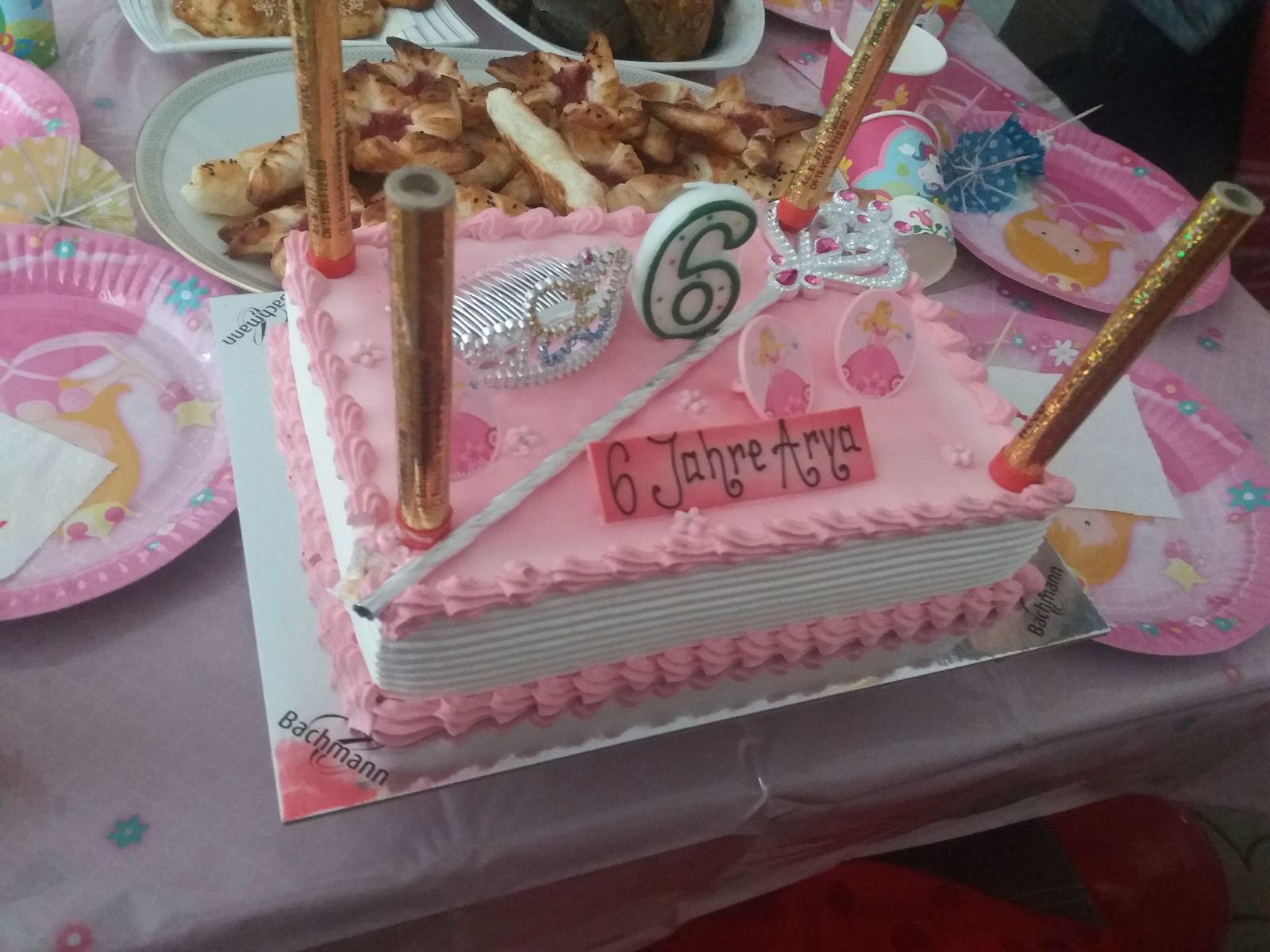This detailed photograph captures a festive scene at a children's birthday party, centered around a beautifully decorated table. Dominating the display is a rectangular birthday cake, adorned with white frosting on the sides and bright pink frosting on top. The cake features a prominent white number six candle bordered with green and topped with green dots, alongside a small silver tiara and a decorative white fairy wand embellished with pink jewels and yellow or white diamonds. Written on the cake in pink frosting is "6 Jahre Aria," which translates to "6 Years Aria," indicating the age and name of the birthday celebrant. Each corner of the cake is marked with golden shimmery cylindrical candles that suggest a potential for a sparkling display.

The table is covered with a white tablecloth decorated with blue and pink flowers, adding to the festive atmosphere. Surrounding the cake are various plates and party items. A central white plate holds croissant-shaped breadsticks, while pink plates featuring the image of a blonde princess in a pink dress holding a star wand are scattered around. The plates also show blue and pink flowers, enhancing the party theme. Additionally, there is a pink cup and a small yellow umbrella visible on the table.

Overall, the photograph beautifully captures the joyful and whimsical atmosphere of Aria's sixth birthday celebration, with its delightful combination of colorful decorations, themed partyware, and delicious-looking treats.